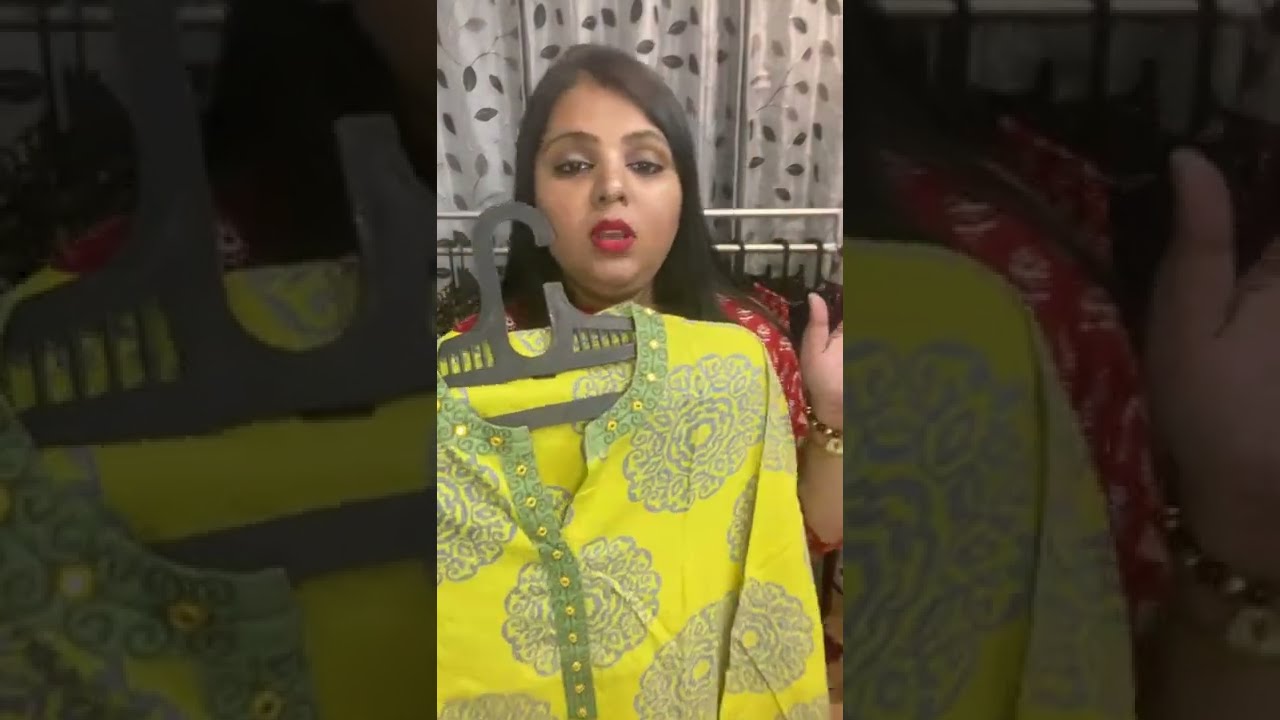The image appears to be a still from a TikTok video, presented in portrait orientation, featuring an Indian woman with long black hair and dark olive skin. She is wearing a red shirt with a white design on it and bright red lipstick. The woman is holding up a yellow shirt adorned with large green and gray floral designs on a black clothes hanger, presenting it to the camera. Her left hand is partially in the frame, palm facing the camera, as if she is gesturing while speaking, which is further indicated by her open mouth and half-closed eyes, possibly caught mid-blink. Behind her is a shiny metal clothing rack filled with various garments, hinting that she might be in a clothing store or her own closet. A black and white curtain is partially visible behind the rack, adding to the ambiguity of the setting, yet suggesting a space dedicated to displaying clothes, reinforcing the impression that she could be selling clothing online through a video.